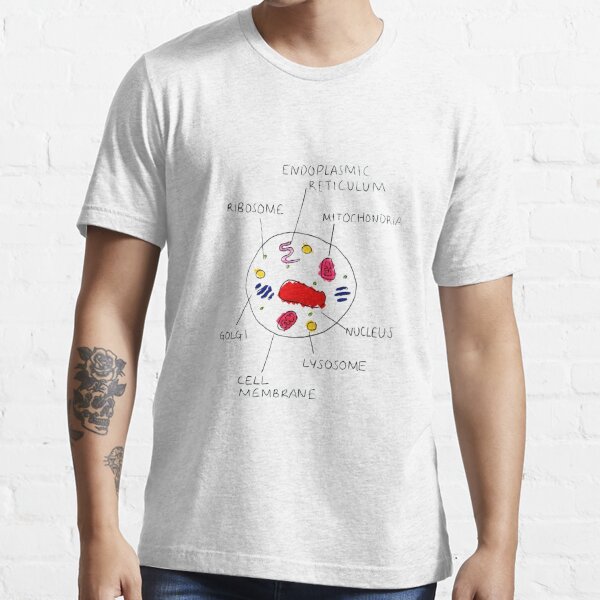The photograph features a man centered in the frame, cut off at the neck and torso, wearing a short-sleeved white T-shirt. The shirt showcases a hand-drawn circular design filled with colored images and black ink labels, depicting cellular structures: ribosome, endoplasmic reticulum, mitochondria, nucleus, lysosome, cell membrane, and Golgi apparatus (mistaken as "gold leaf"). His bare arms hang at his sides, revealing partial views of his hands and tattoos. On his right forearm, a tattoo of a skull with a rose above it is visible, along with another tattoo near his wrist, partially seen. Beneath the T-shirt, a glimpse of his blue jeans is visible. The background consists of white-painted brick, enhancing the image's detail and contrast.